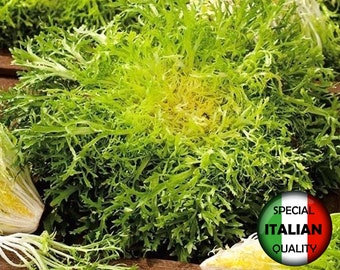A vibrant, real-life image showcases an abundant cluster of fresh arugula, occupying the majority of the scene. The leaves, with their distinct arugula appearance, radiate from a central focus where shades of dark and light green intermingle. The central portion, particularly facing the camera, reveals lighter green hues and a subtle whitish-green core. Surrounding the arugula, various vegetables are partially visible adding texture and complexity to the image. To the bottom left corner, a small bunch resembling Brussels sprouts can be noticed, while the bottom right corner reveals what seems to be the base of a celery. A circular object, resembling a pin, is discernible with shadows that create a three-dimensional effect. The backdrop of the image consists of horizontal stripes in green, white, and red, reminiscent of the Italian flag. Superimposed on this tricolor background is a bold, black text stating: "SPECIAL" at the top, "ITALIAN" in prominent letters in the middle, and "QUALITY" at the bottom.